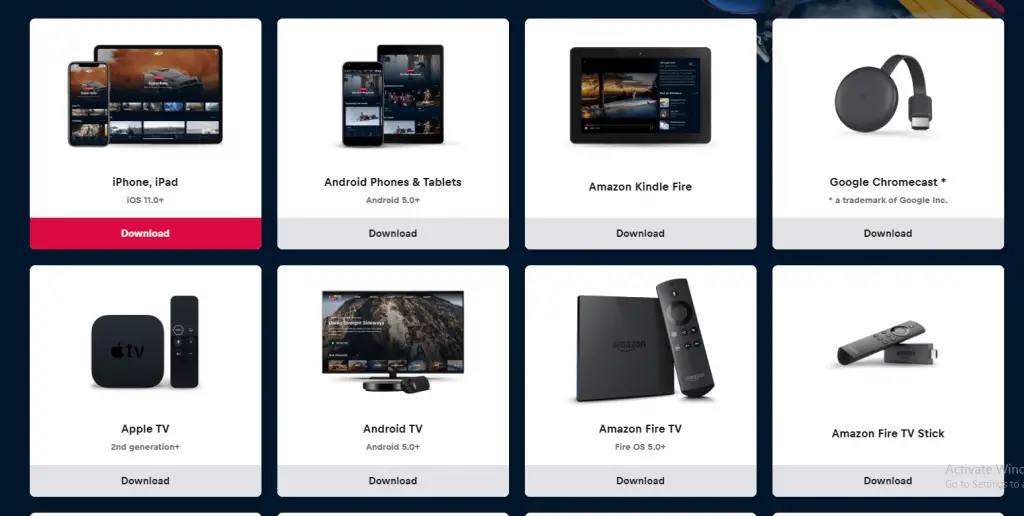The image is a square with a black background, segmented into eight even-sized boxes arranged in a 2x4 grid. Each box represents a different platform and provides information for downloading its respective application.

- **Top Left Box**: This box features icons of an iPhone and an iPad, labeled "iPhone, iPad." The download button is highlighted in red, indicating that you can click it to download the application for these devices.
- **Top Second Left Box**: Titled "Android Phones & Tablets," this box displays a download button for devices running Android 5.0 or higher.
- **Top Third Left Box**: Specifically for "Amazon Kindle Fire," this box provides a download option for the Kindle Fire devices.
- **Top Right Box**: The box shows the "Google Chromecast" with a trademark of Google Inc. Users can click the download bar to get the application for Chromecast.

On the bottom row:

- **Bottom Left Box**: Labeled "Apple TV Second Generation Plus," this box includes a download bar for compatible Apple TV devices.
- **Bottom Second Left Box**: Named "Android TV," this box exhibits an image of a television set with a mountain outline and offers a download option for devices with Android 5.0 or higher.
- **Bottom Third Left Box**: This box is for "Amazon Fire TV" and includes a download button for devices with Fire OS 5.0 or above.
- **Bottom Right Box**: Featuring the "Amazon Fire TV Stick," this box provides an image of the device and a download option.

Each download button in these boxes ensures easy access to the corresponding applications for each specific device or platform.